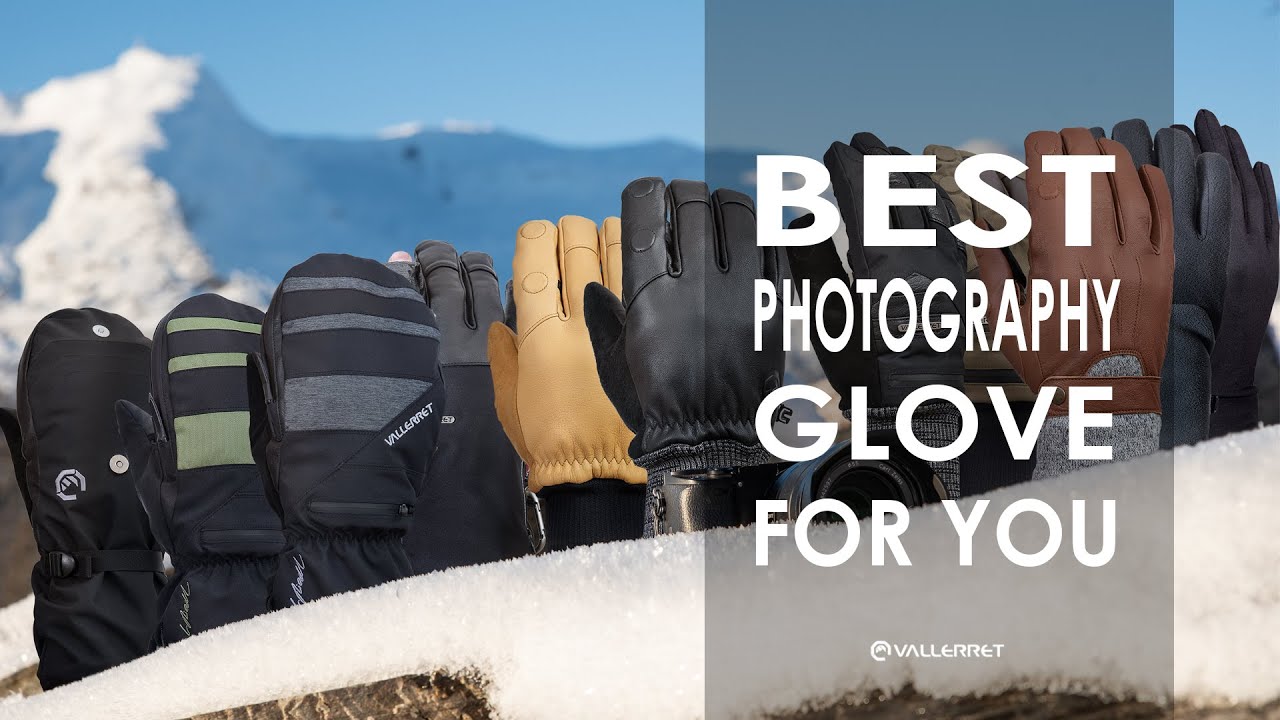The image is a detailed advertisement for Valorette, a company specializing in photography gloves. It features approximately a dozen gloves, each uniquely designed, positioned upright on some kind of mannequins aligned in a row that almost evokes the iconic Stonehenge formation. The gloves, varying from fingerless to full mittens, display different colors and patterns, with most being darker shades and one notably bright yellow. Positioned against a wintry backdrop with a slightly out-of-focus snowy mountain peak and a clear blue sky, the scene emphasizes the outdoor, cold-weather utility of the gloves. An icy-covered rock sits prominently in the foreground. Overlaying the top right of the image is the text "Best photography glove for you" in vertical white letters, with the brand name "Valorette" in smaller font at the bottom on a transparent dark stripe.